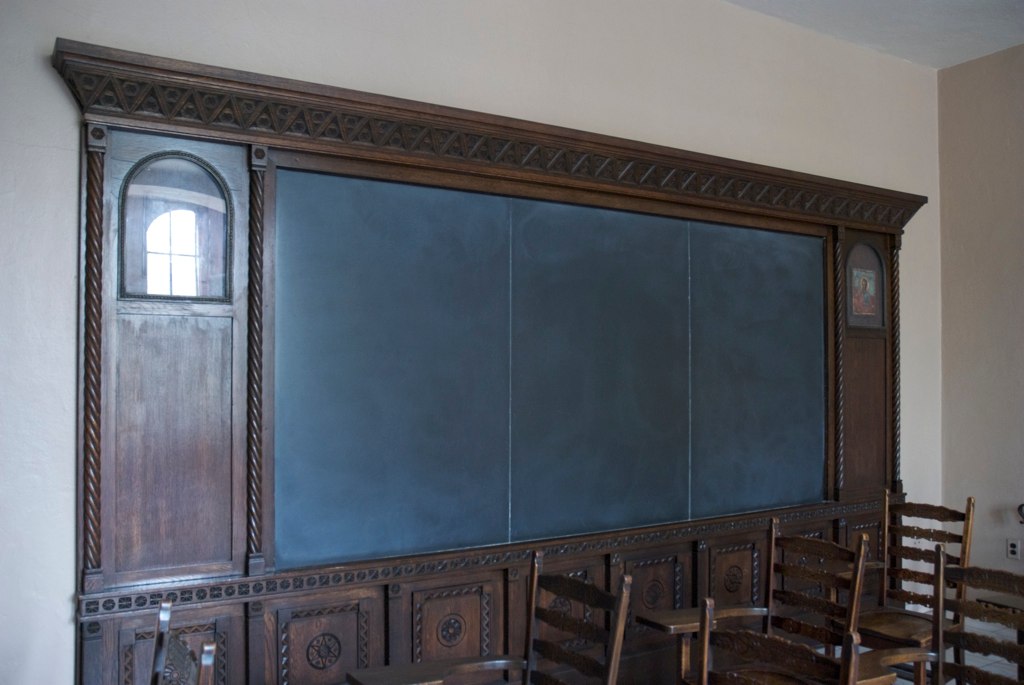The image depicts a color photograph of an old-fashioned classroom with a sidewall designed to evoke a sense of status and elegance. The walls are painted beige, and a corner of the white ceiling is visible in the upper right corner. The focal point of the wall is a central section adorned with dark wooden paneling featuring intricate braided etchings and build-outs, reminiscent of Victorian design. This elaborately decorated wooden structure houses three large, spotless blackboards framed by clear arch-topped glass panels on either side. Beneath these, there are multiple wooden panels and likely some shelving units.

In front of this detailed wooden setup are five vintage wooden student desks, although more are likely present off-frame. These desks are connected to chairs, each with a right-side armrest that serves as a writing surface, characteristic of old-time classroom furniture. The room appears to be naturally lit, as there are no visible light fixtures, with reflections of windows seen on the glass panels. Overall, the scene combines the historical elegance of the wooden decor with the functional simplicity of an educational setting.